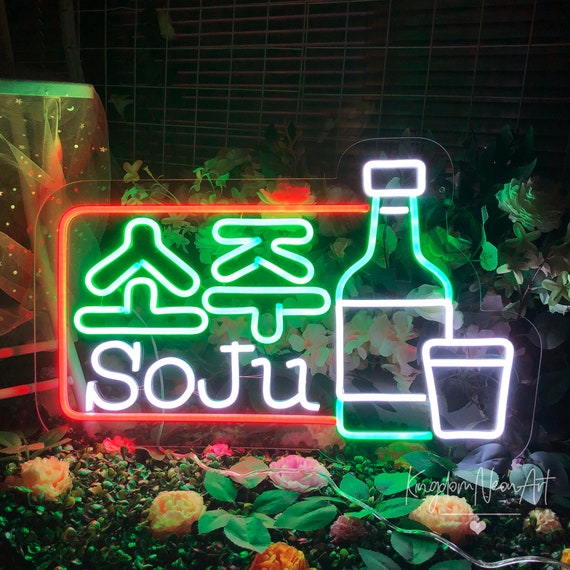The photograph captures a striking neon sign, featuring a red border and the word "SOJU" prominently displayed in white at the bottom. Above this, there are Korean characters that resemble an upside-down Y, an upside-down T, an upright T, and another indistinct symbol. To the right of the word "SOJU," there is a detailed depiction of a green bottle with a white label and cap, accompanied by a smaller white cup at its base. The vivid sign seems to illuminate a lively scene, as it is surrounded by an arrangement of green plants and colorful flowers in shades of pink, yellow, and orange. On the left-hand side of the image, an aquarium-like structure with bubbles ascending and what appears to be kelp inside adds another layer of interest. The background is dark, enhancing the neon glow of the sign, which is also marked with a watermark reading "Krypton Neon Art" in a stylized script in the bottom right corner. The combination of light and color suggests this could be a piece of art or an advertisement perhaps for a bar or similar establishment.